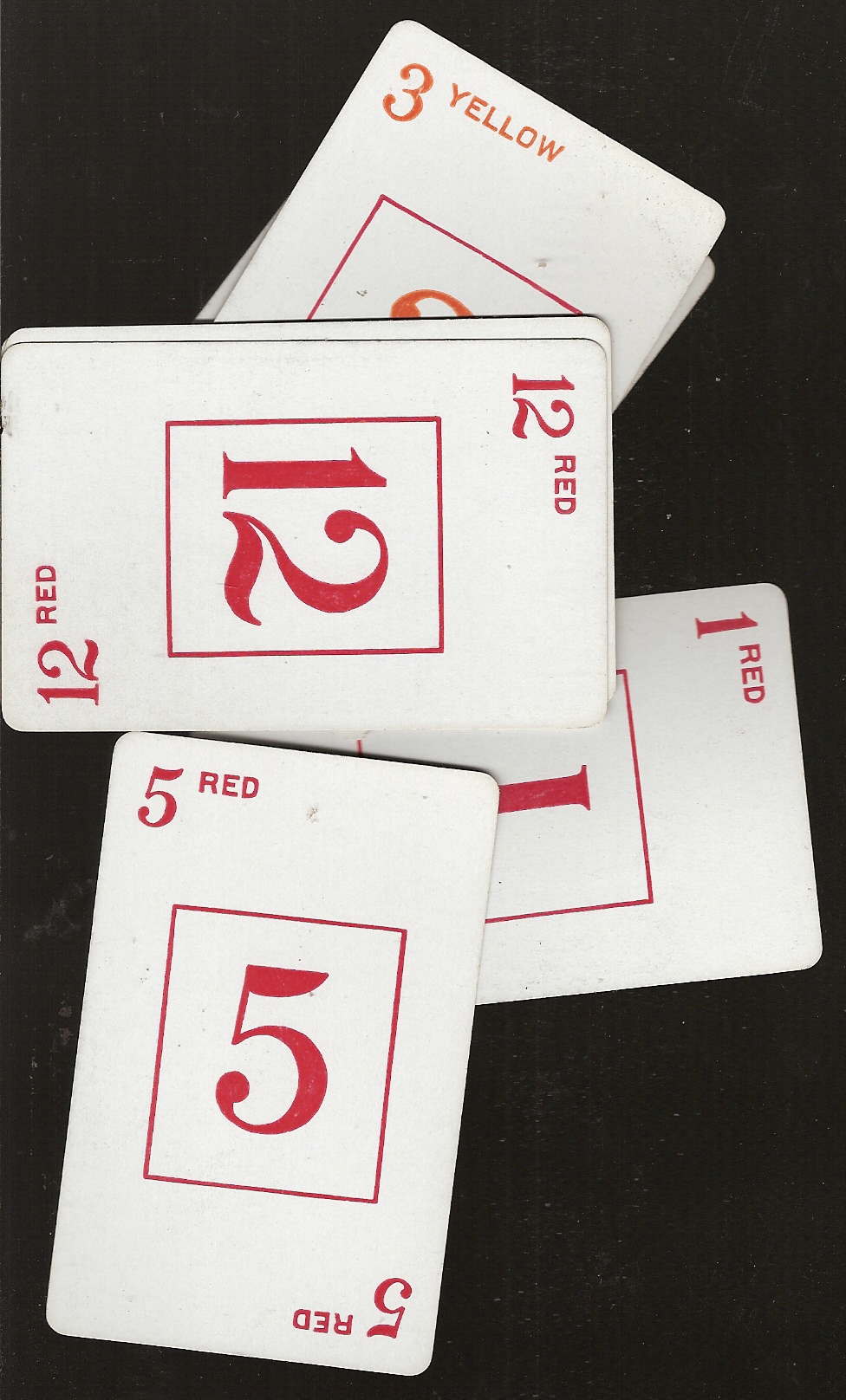This detailed aerial photograph showcases a dark-colored table with a subtle textured pattern of lines. Positioned from top to bottom, there are two cards stacked closely together at the top. The top card prominently displays the number "3" and the words "three yellow," although the color appears slightly orange. It features a central square outlined in red, with a bold "3" in its center. Barely visible beneath this card is another, whose details are obscured.

Perpendicular to the frame, two additional cards are aligned, with one card partially concealing the other. The more visible card displays "12 red" with a square in the center, containing a bold "12." This card's bottom left corner also shows "12 red" in typical playing card style. Underneath these, slightly angled back towards the left, is a "1 red" card. Overlapping vertically atop this "1 red" card is a "5 red" card, leaning subtly to the right. 

The meticulous arrangement and details of these colorful cards against the textured dark surface create a visually engaging composition.